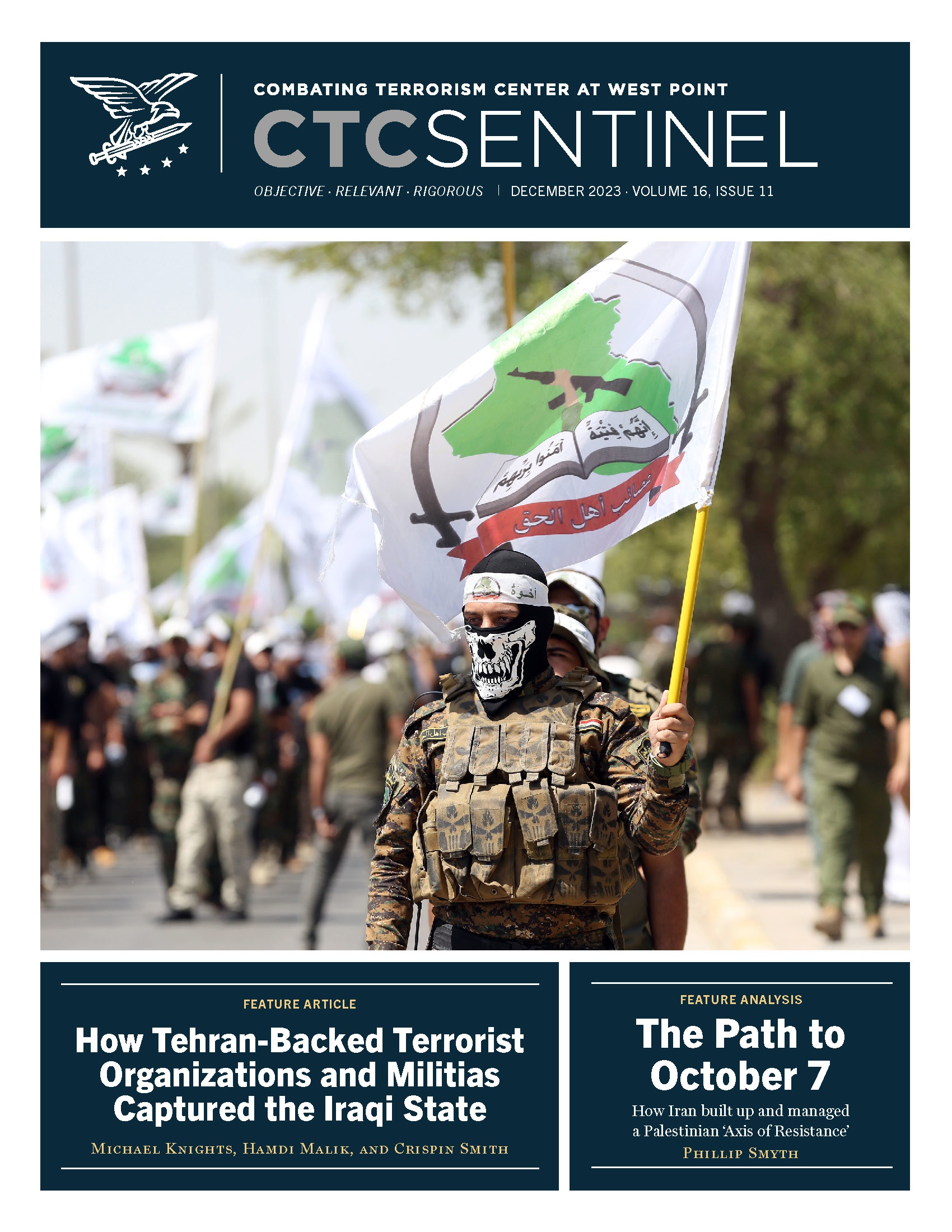This image depicts a vertical, rectangular flyer or poster with a detailed layout. At the top, within a dark blue horizontal rectangle, white text reads: "Combating Terrorism Center at West Point CTC Sentinel," followed by "Objective, Relevant, Rigorous," and "December 2023, Volume 16, Issue 11." To the left of this text is a logo featuring an eagle carrying a sword, with four stars beneath it.

Below this header, a central photograph shows a group of soldiers, some in khaki and camouflage outfits, and one prominently focused soldier wearing camouflage and a black face mask with a skull design. This soldier is holding a white flag with Arabic writing, images of a sword, a green country profile, and a book. The flag is on a yellow stand, and the background includes blurred figures, some appearing to be protesters or additional soldiers carrying similar flags.

At the bottom of the image are two dark blue rectangles with white text. The left rectangle reads: "Feature Article: How Tehran-Backed Terrorist Organizations and Militias Captured the Iraqi State," credited to Michael Knights, Hamdi Malik, and Crispin Smith. The right rectangle states: "Feature Analysis: The Path to October 7th, How Iran Built Up and Managed a Palestinian Axis of Resistance," penned by Philip Smith.